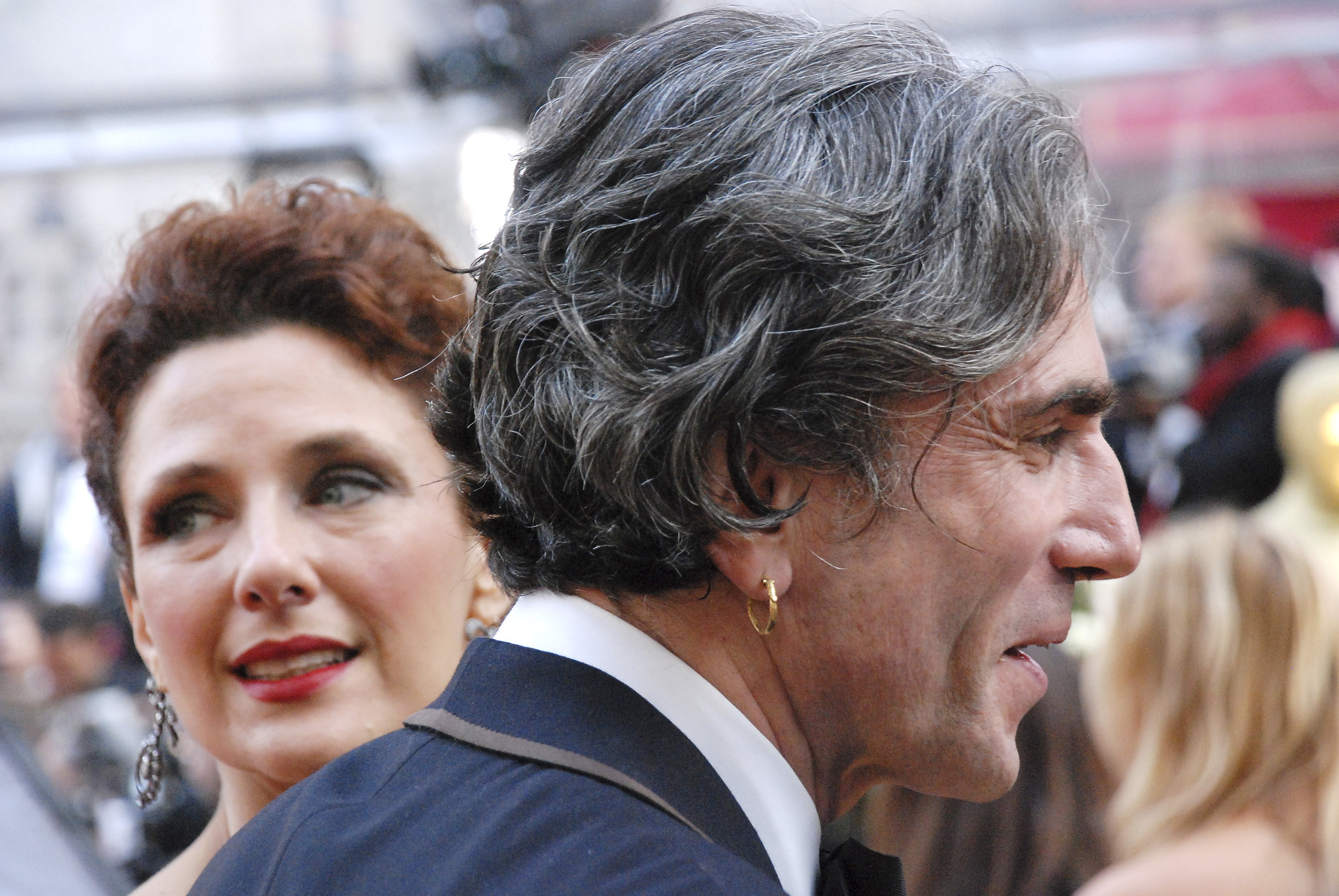In this detailed, landscape-oriented color photograph, the primary focus is a side profile of an older Rick Springfield. He looks to the right, mouth open as if speaking to someone just out of frame. Wearing a blue blazer and a white collared shirt, he also sports a gold hoop earring in his right ear. His hair is mostly gray with hints of black, mid-length and slightly tousled. Beside him, a woman with dark reddish-brown hair, adorned with blue eyeshadow and red lipstick, looks leftwards. She has on long, dangly, sparkly earrings. The background features a blurred crowd, hinting at a public event or gathering, possibly outside given the bright lighting. There's an impressionistic realism in the representation of the scene, capturing both the individuals and the ambiance around them with an almost lifelike clarity.